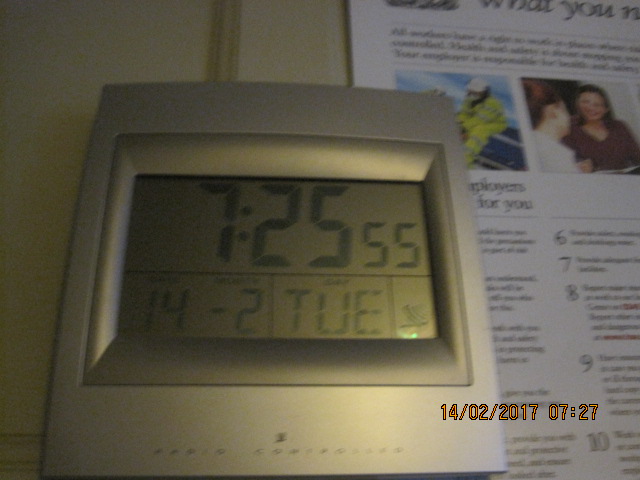The image depicts a dark setting with a large silver symbol prominently displayed against a white background. Central to the image is a digital clock, slightly to the left, featuring black numerals on an LCD display. The time on the clock reads 7:25:55, and beneath it, the day is indicated as "TUE," alongside the date "14-2." To the right of the clock, there appears to be a brochure or magazine with pictures of two women facing each other, visible in color. The brochure contains numbered columns and paragraphs, though the details are blurred and unreadable. In the bottom right corner of the image is a timestamp, marking the date as February 14th, 2017, at 07:27, mirroring the time on the clock.